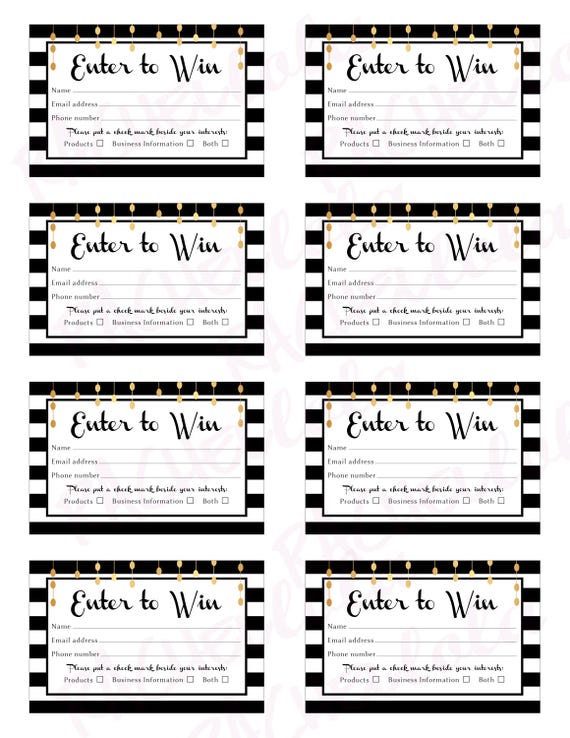This photograph depicts an 8 1/2 by 11-inch sheet, likely intended for cutting into smaller, individual contest forms or raffle tickets. The sheet is organized into two rows of four, making a total of eight identical sections. Each segment features a black and white striped border with gold-colored pendent designs at the top, adding a decorative touch. Dominating the center of each section is the phrase "ENTER TO WIN" written in cursive. Below this, there are three labeled lines for participants to fill in their NAME, EMAIL ADDRESS, and PHONE NUMBER. Further down, there's a statement instructing participants to "PLEASE PUT A CHECKMARK NEXT TO YOUR INTEREST," accompanied by three options: PRODUCTS, BUSINESS INFORMATION, and BOTH, each with a corresponding box to check. This appears to be a marketing tool designed to attract and gather leads, possibly offered as a digital download template with a faded background to prevent unauthorized use.